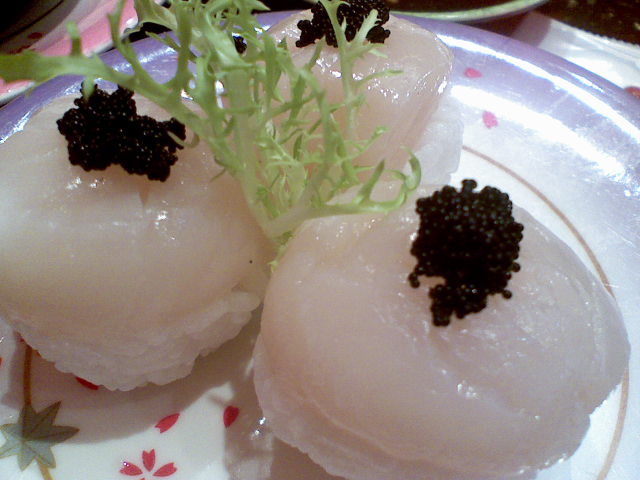The image depicts a close-up of an elegant sushi dish, featuring three pieces of nigiri artfully arranged in a triangular formation on a decorative plate. Each piece of nigiri consists of a small bundle of sticky white rice topped with a glossy slice of white-fleshed fish, adorned with a small dollop of black caviar or roe. At the center of the three nigiri pieces, a sprig of light green baby lettuce serves as an eye-catching garnish, reminiscent of an underwater coral. The plate itself boasts a white background with a purple rim and is embellished with a vibrant pattern of green leaves and red flowers. Surrounding the main plate, the edges of other colorful bowls can be seen, suggesting a setting in a high-end restaurant.